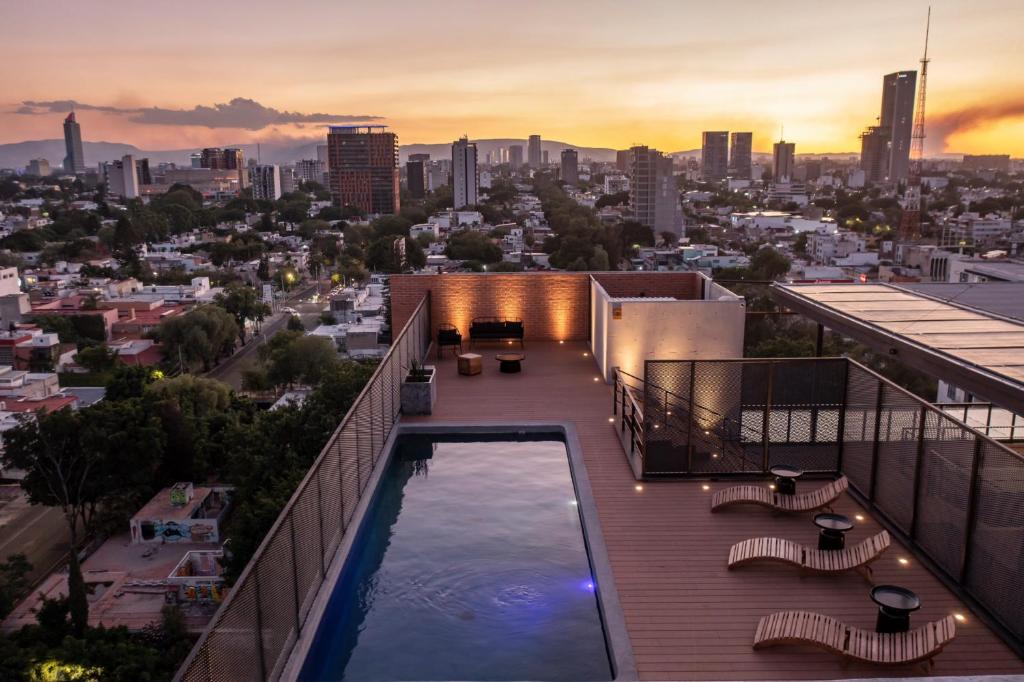This photograph captures an outdoor rooftop pool area of a building, likely an apartment complex. In the center of the image, a serene pool surrounded by a wooden deck is featured prominently. Curved, wooden sunbathing chairs line the sides of the pool, each accompanied by a small black table, creating a comfortable setting for relaxation. The pool deck is equipped with track lighting along the floor, enhancing the ambiance during twilight hours. To the left of the pool, a glass fence wall provides security, while the right side of the rooftop includes an elevated loft area with additional seating on a short brick-walled section, leading down to a covered area with a set of descending stairs. 

The backdrop showcases a sprawling cityscape with scattered skyscrapers visible towards the left, center, and far right. Low-rise white and red buildings intermingle with dense tree lines and streets, contributing to the city's greenery. A noticeable radio tower antenna stands tall on the right. The photograph was taken during a picturesque sunset, illuminating the sky with bright yellow and pink hues, casting a glowing light over the urban landscape.